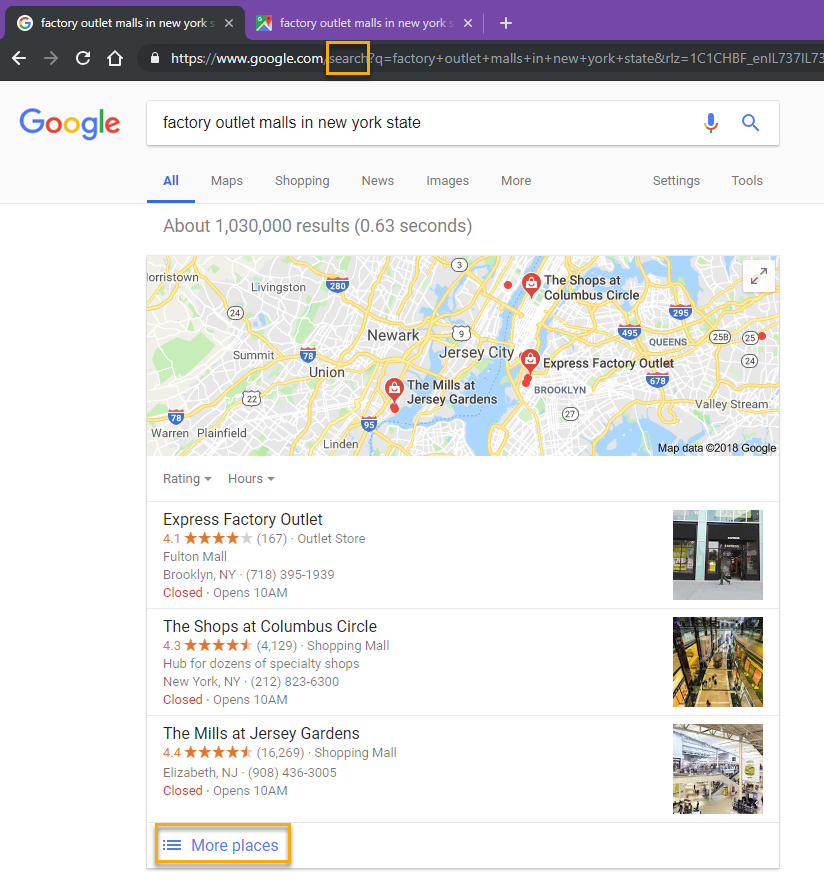The image is a screenshot from a Google search for "factory outlet malls in New York State." At the top of the image is a purple navigation bar with black lower accents, indicating the search interface. Below this navigation bar, the actual search results are displayed.

The first notable element is a title in a prominent box, stating "Factory Outlet Malls in New York." Beneath this title is a detailed map pinpointing three specific outlets. Each pin is associated with one of the following locations: 

1. **Express Factory Outlet** in Brooklyn, New York.
2. **The Shops at Columbus Circle** in New York, New York.
3. **The Mills at Jersey Gardens** in Elizabeth, New Jersey.

Next to each pin on the map, there are thumbnail images providing a visual reference for what each outlet mall looks like.

Below the map, there is a gold-colored box with blue text reading "More places." This box contains horizontal lines that presumably can be clicked to reveal additional factory outlet malls for shopping in the broader area.

The map itself not only shows New York City but also extends to parts of New Jersey and Queens, highlighting the geographical spread of the search results beyond just the immediate city area.